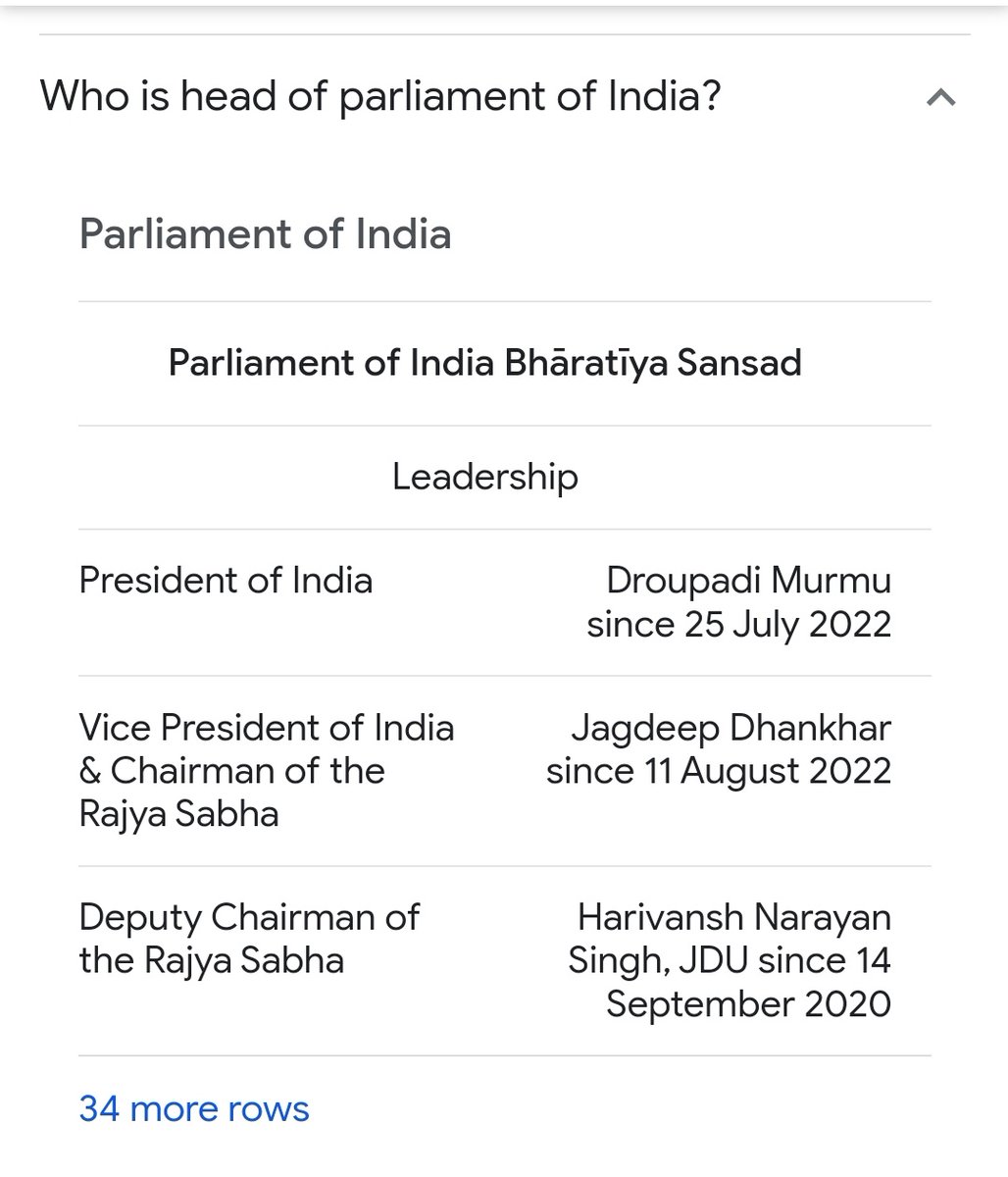The image is a clear and easy-to-read screenshot of a search results page on a white background. At the top, the query reads, "Who is head of Parliament of India?" Below this is the heading "Parliament of India," repeated once, followed by an Indian name which appears to be unidentified in the description. Further down, under the subheading "Leadership," there are three distinct rows outlining key positions within the Indian Parliament: 

1. The left side of the first row states "President of India," with the President's name and the note "since 25 July 2022" aligned to the right.
2. The second row specifies "Vice President of India and Chairman of the Rajya Sabha," with the corresponding name and date "since 11 August 2022" on the right.
3. The third row indicates "Deputy Chairman of the Rajya Sabha," followed by a name and the date "since 14 September 2020" on the right.

At the bottom of the list, in blue clickable text, is the option "34 more rows." All text except this clickable link is in black, using a large font that enhances readability. There are no other colors, images, or objects present in the screenshot.